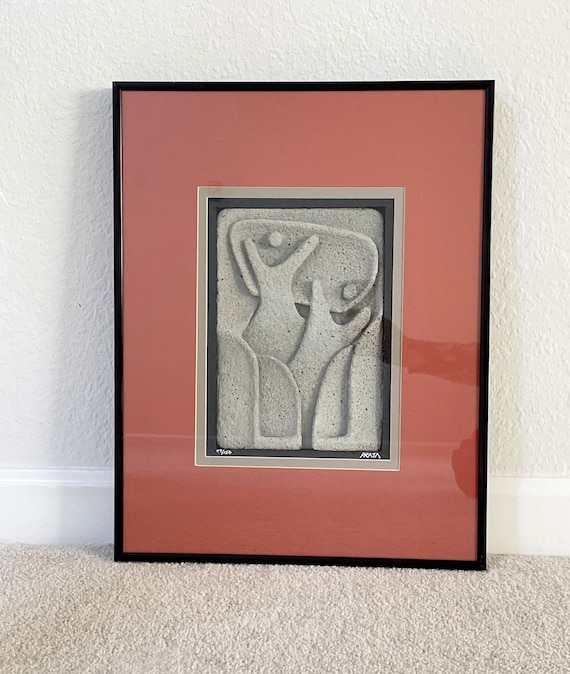The image depicts a framed abstract art piece positioned on a white, carpeted floor, leaning against a white wall. The artwork is encased in a sleek black frame, which encompasses a broad matte border of a reddish-tan or dark pink hue. Within the center of this matting lies the main art piece, characterized by an abstract, stone-colored design that incorporates various shapes and figures. Notably, there appear to be two prominent, wide Y-shaped humanoid figures, each with a central dot at the top, symbolizing heads with raised arms. Beneath these figures, there is a series of similarly abstract, arch-like forms that could be interpreted as either curled structures resembling tacos or interconnected arched monoliths. The wall behind the art is white, matching the crown molding at the bottom, and the floor beneath the piece features a brown carpet, adding contrast to the otherwise monochromatic background.